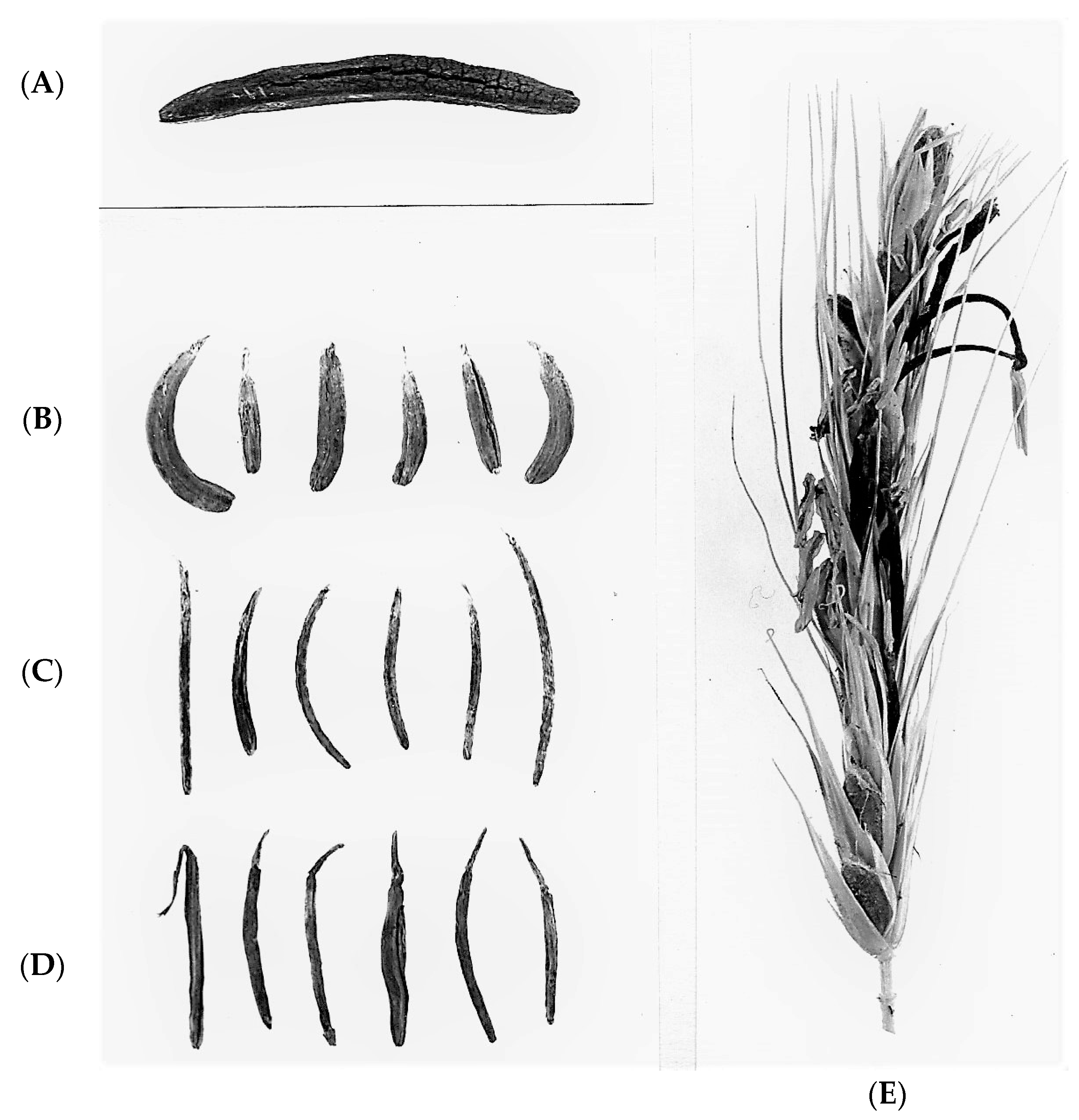This black and white diagram consists of five distinct elements labeled A through E, showcasing different brush strokes and a plant illustration. On the left side of the image, there are four sections labeled A, B, C, and D in parentheses, positioned vertically from top to bottom. The brush strokes include:

- **A**: A thick, worm-shaped, solid black stroke.
- **B**: Six lined-up cylinder shapes resembling short pickles, dark and varied in sizes.
- **C**: Six curved, thick black lines of differing lengths and sizes.
- **D**: Six thin, pepper-shaped strokes with slimmer tips, uniformly aligned but varied in length.

To the right, labeled **E**, is a detailed illustration of a tall, stocky plant, possibly wheat or corn, characterized by its many wispy, straw-like extensions. The plant has thin, vertical elements with a prominent stem and what appears to be white petals or leaves that seem wilted.

The diagram is detailed without scientific notations, enhancing the visual differentiation and characteristics of each brush stroke and the plant illustration.